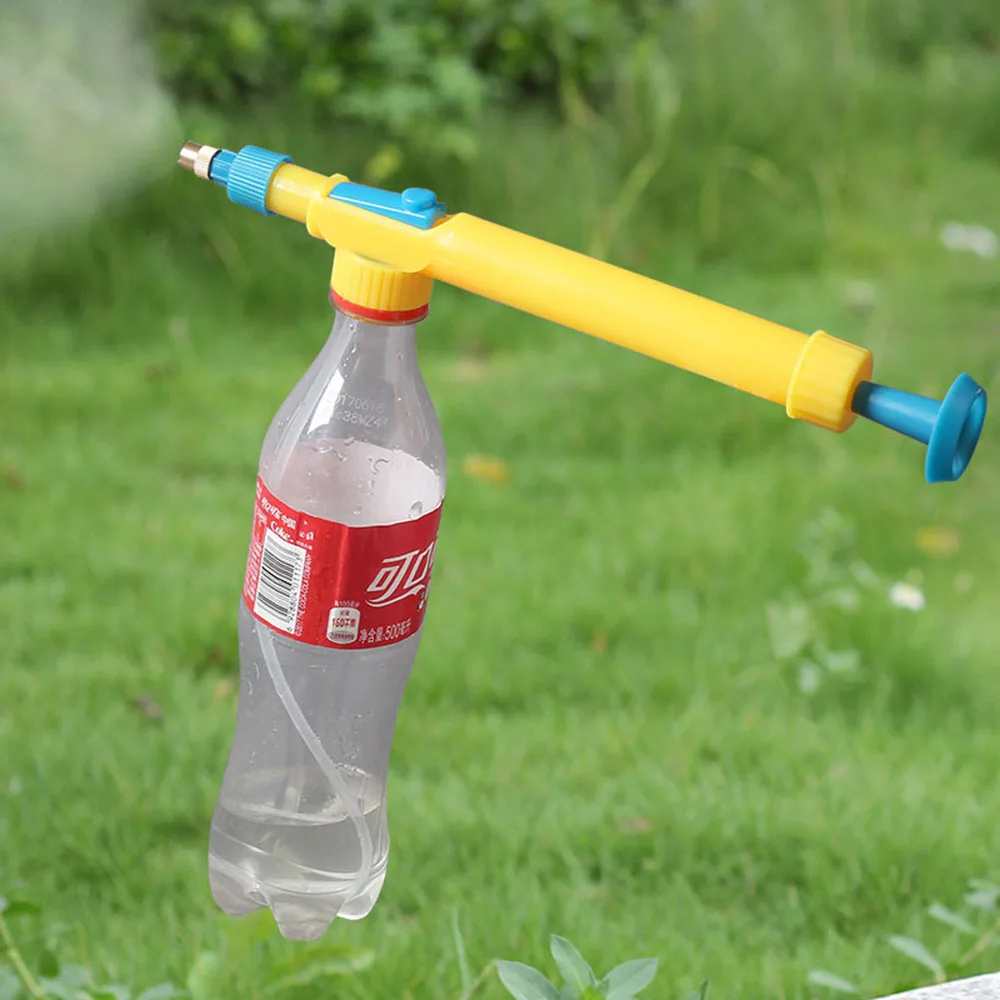The image features a converted soda bottle with a clear body and a red label, resembling a 12 or 16-ounce bottle. The bottle has a distinctive attachment that transforms it into a misting device. This yellow cylindrical attachment screws onto the bottle's cap and includes a blue plunger on one end and a spout with a silver metal tip on the other. Inside, a tube extends down into the bottle, which contains a translucent liquid. The device appears to be in use, with mist visibly spraying from the spout. The bottle is positioned lying on its side in a grassy area filled with green grass, scattered leaves, and light-colored flowers. The background is a blur of taller grass and plants, suggesting the image was digitally placed onto this scenic backdrop.